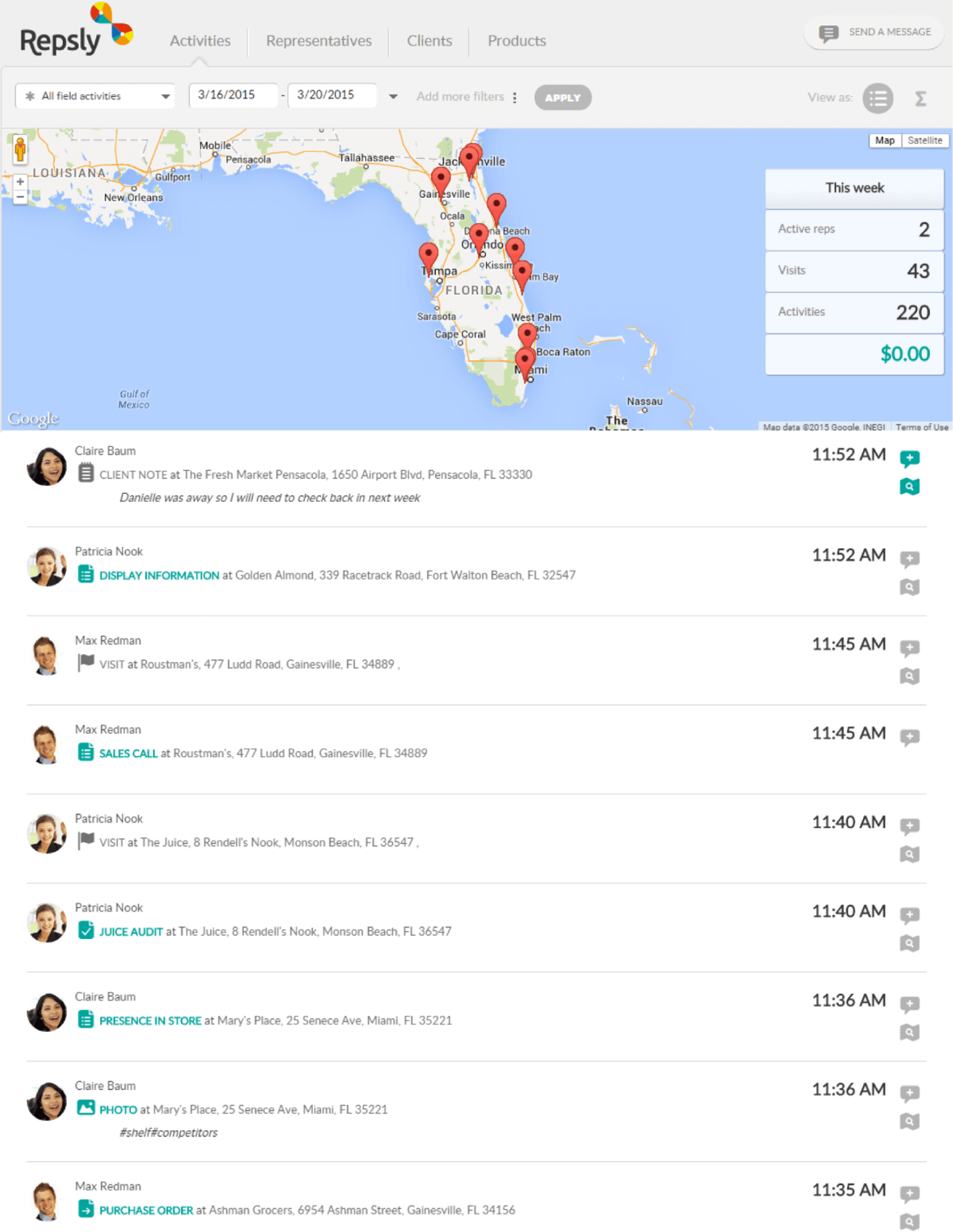The website for Repsly is prominently displayed with the company name in the upper left corner. Adjacent to it are navigation options labeled: "Activities," "Representatives," "Clients," and "Products." Directly below, a timeline is indicated for all field activities dated from March 16 to March 20, 2015.

A detailed map, predominantly featuring Florida, serves as the centerpiece. It is dotted with numerous reddish-orange pins marking significant locations. Notable cities such as Sarasota, Cape Coral, Ocala, and Tallahassee are clearly labeled. Additionally, the map extends to show a glimpse of Louisiana with cities like New Orleans marked.

To the right of the map, a section titled "This Week" provides a summary:
- Active Reps: 2
- Visits: 43
- Activities: 220
- Revenue: $0.00

Below this, there's a profile featuring an icon of a woman with the name "Claire Baum." Her client note at the Fresh Market in Pensacola reads: "Danielle was away, so I will need to check back in next week," followed by the address.

Successive profiles include:
- Patricia Nook, twice represented by an icon.
- Max Redman, appearing once with a picture and once more with another image.
- Repeat appearances of Patricia Nook and Claire Baum, each shown in subsequent images.

The final image again features Max Redman, rounding off the visual documentation of the representatives' activities for the week.